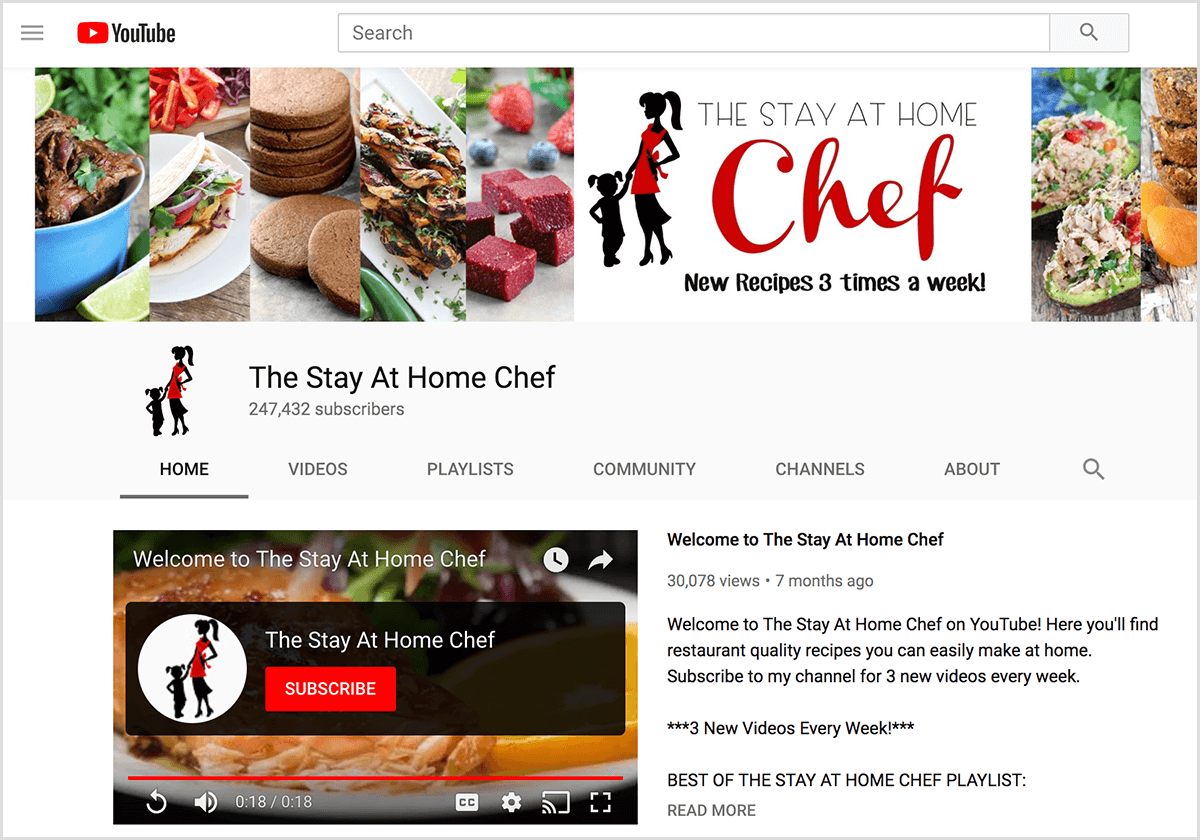This image is a screenshot from the YouTube channel "The Stay-at-Home Chef." The YouTube logo is prominently displayed in the upper left-hand corner against a clean, white background with black text. The channel's banner features the cartoon logo of a woman and a child, both with black hair and simple, stylized facial features. The woman is depicted wearing a red tunic and a black skirt, with her hair in a ponytail, while the child, whose entire body appears black, has pigtails.

The text "The Stay-at-Home Chef" is prominently written in black, with the word "Chef" standing out in red. On either side of the logo, there are images of mouth-watering dishes, emphasizing the culinary theme of the channel. The channel boasts 247,432 subscribers, and the "Home" tab is currently selected, with other tabs such as Videos, Playlists, Community, Channels, and About also visible, along with a search button.

Below the main banner is a featured video titled "Welcome to The Stay-at-Home Chef," which has garnered 30,078 views in seven months. The text beside the video reads, "Welcome to The Stay-at-Home Chef on YouTube. Here you'll find restaurant-quality recipes you can easily make at home. Subscribe to my channel for three new videos each week." There's also a "Subscribe" button visible under the video preview, alongside a thumbnail image of a delicious meal. Additionally, there is a note about the "Best of The Stay-at-Home Chef" playlist, accompanied by a "Read More" prompt.